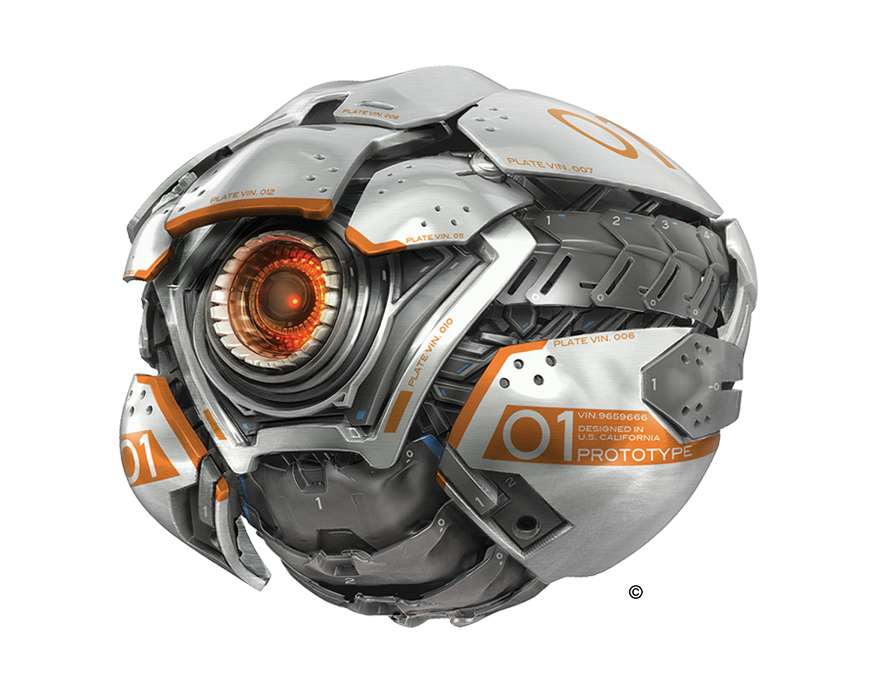The image depicts a highly futuristic, metallic drone or robot, designed with an aesthetic reminiscent of a robotic head. Its body is predominantly dark black and light silver metal, adorned with striking orange highlights. Central to the design is a singular eye-like feature, resembling a round, red-tinted lens with orange lights emitting from within, giving it a lifelike appearance. This eye is flanked by vertical white pieces, possibly part of a protective shutter mechanism. The structure includes several overlapping plates, particularly noticeable atop the eye in two groups of three and around the circular head, with distinct orange stripes highlighting its contours.

On the bottom portions, detailed orange stripes bear white inscriptions, including a prominent "01" and smaller text reading "Designed in U.S. California, prototype". Additional writing and interlocking gray metal pieces are observed atop the head, adding to the intricate details of the mechanism. The design suggests potential versatility, where the device might unfold to reveal its sensor and possibly perform various functions like filming, emitting light, or even projecting a laser, before closing back into its streamlined form. The overall design and color scheme evoke a strong resemblance to advanced tech seen in science fiction, such as in Star Wars.